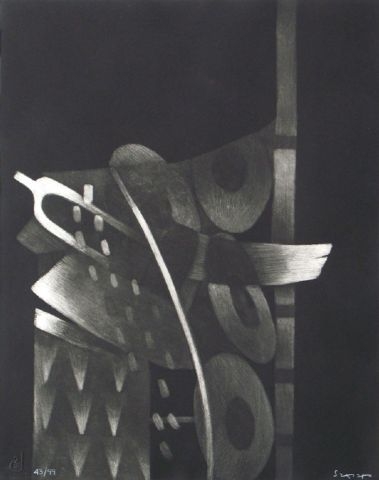The image is a dark, abstract artwork with a predominantly black background. Centered and descending from the middle is a prominent white, curved line. To the left of this line are several upside-down triangular shapes, each featuring a white tip and a gray base. The right side of the curving line includes multiple gray circles, each containing a small black center. The bottom right contains white, somewhat indistinct writing. The piece appears to combine computer-generated elements or pencil drawing techniques, with shading that suggests various shapes, including what resembles the number zero and layered forms, creating a textured, dynamic composition. The top right is dominated by dark gray hues, interrupted intermittently by stark black shades, creating a sober, layered visual effect.